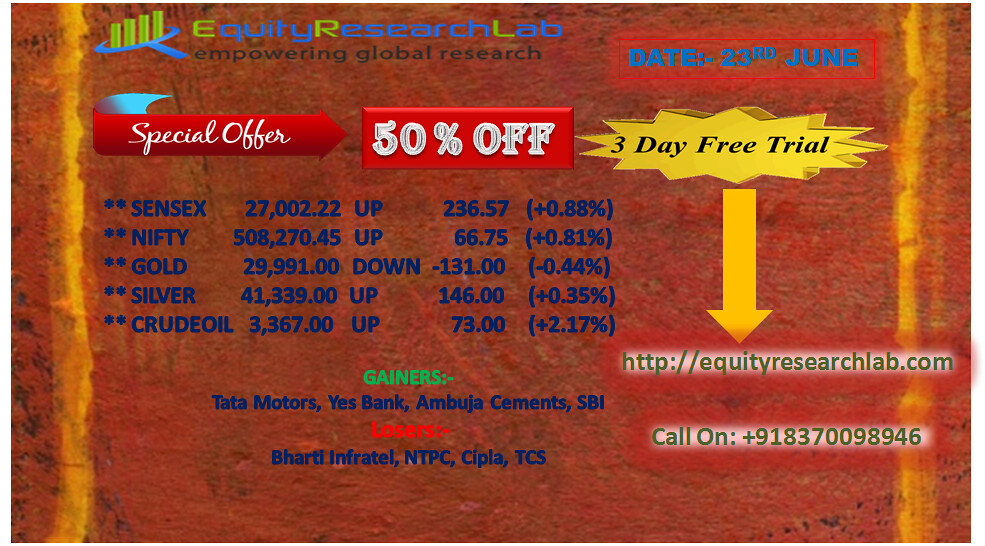The advertisement poster for Equity Research Lab, featuring the tagline "Empowering Global Research," prominently displays the company's logo in the top left-center in blue and green. Dated June 23rd, the poster highlights a "Special Offer" in red, boasting "50% Off" in bold text. A yellow graphic box announces a "Three-Day Free Trial," pointing to the website, equityresearchlab.com, and provides a contact number, 918-3700-98946.

The central portion of the poster, set against a red background with yellow vertical stripes on the sides, showcases examples from various markets, including Sensex, Nifty, Gold, Silver, and Crude Oil. It presents the predicted upticks and downticks along with specific numeric values to illustrate percentage changes. The poster also emphasizes the firm's successful track record with gainers such as Tata Motors, Yes Bank, Abuja, Semence, and SBI, while listing some of the losers like Beharty, Infratel, NTPC, CIPLA, and TCS. Overall, the poster serves as a detailed and persuasive advertisement for the firm's equity research services.